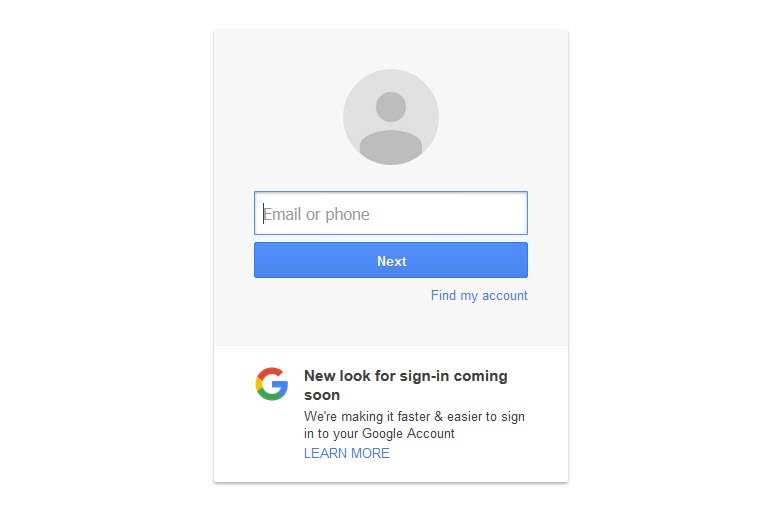This image depicts a vertical, narrow, and sparsely populated Google sign-in screen on a phone. At the top of the screen, there's a circular icon with a small gray person figure inside, symbolizing Google’s user profile placeholder. Directly beneath this icon is a search box that provides two options: "Email or phone," indicating where users can input their credentials. The search box is followed by a bright blue button labeled "Next" in white font, guiding users to proceed with the sign-in process.

Below the “Next” button, there is a line of blue text stating "Find my account," offering additional assistance for account recovery. Towards the bottom, there is a rectangular area containing the multicolored Google logo, accompanied by a message informing users of an upcoming change: "New look for sign-in coming soon." This announcement is followed by the text, "We're making it faster and easier to sign into your Google account," describing the purpose behind the forthcoming redesign. Finally, in blue, capitalized letters, the text "LEARN MORE" invites users to read further details about the update.